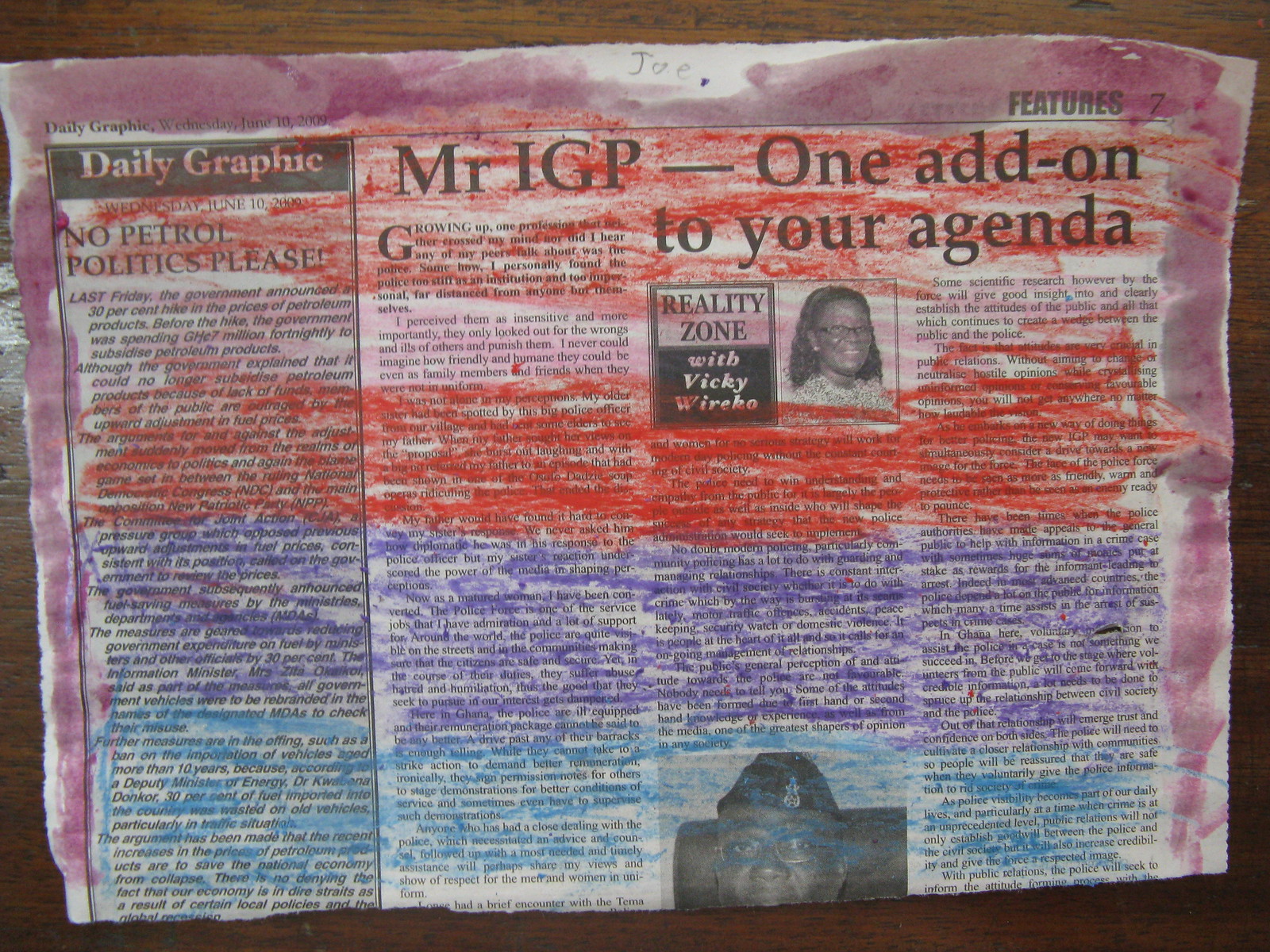This rectangular image, approximately 6 inches wide by 5 inches tall, depicts an old newspaper article placed on a brown wooden surface. The article, which is primarily black and white, appears to be the upper half of a newspaper page and is bordered with purple-pinkish paint. Prominent text at the top reads "Daily Graphic - No Petrol Politics Please Mr. IGP: One Add-on to Your Agenda." Below this headline, a picture of a young woman titled "Reality Zone with Vicki Weirich" is visible. The bottom of the image also features a man wearing a hat. The newspaper has been extensively colored over with crayons, obscuring much of the text. The crayon markings form a series of horizontal stripes: a red stripe at the top, followed by layers in pink, dark red, purple, and blue. These vibrant layers render much of the newspaper's original content unreadable.